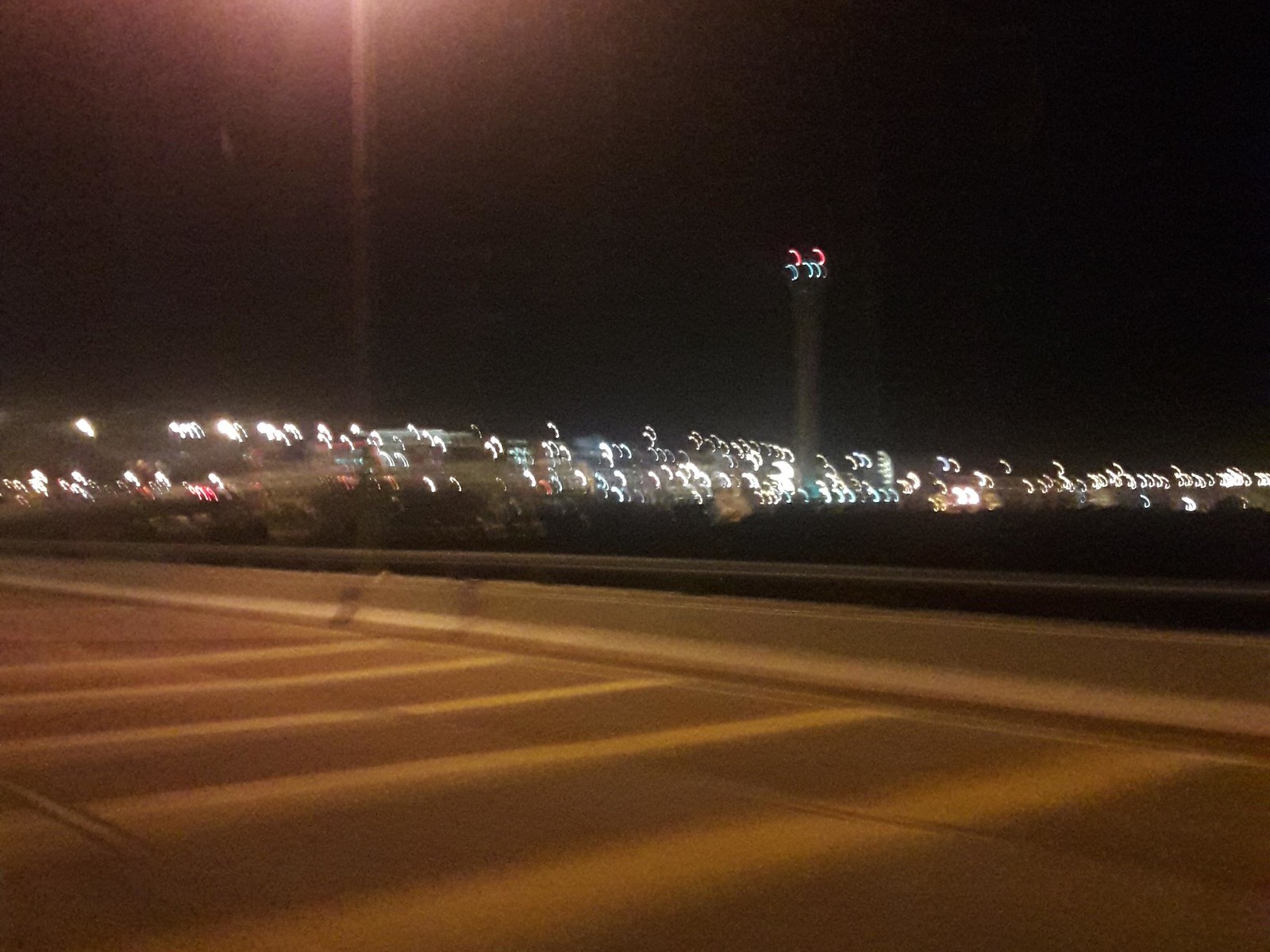A nighttime scene captured in a very blurry photograph, where the bottom half is dominated by gray pavement. A thick white line runs horizontally across the center, slightly slanting towards the right. From the left side, several vertical lines, which appear to be yellow despite the blurriness, intersect the white line. Beyond it lies a road, bordered by a gray guardrail. Past the guardrail, there's a dark area leading out to a distant, softly illuminated cityscape with muted lights. At the center stands a tall gray tower crowned with red and white lights. Topping the image is a dark sky, punctuated by a conspicuous circular reddish light in the upper left corner.